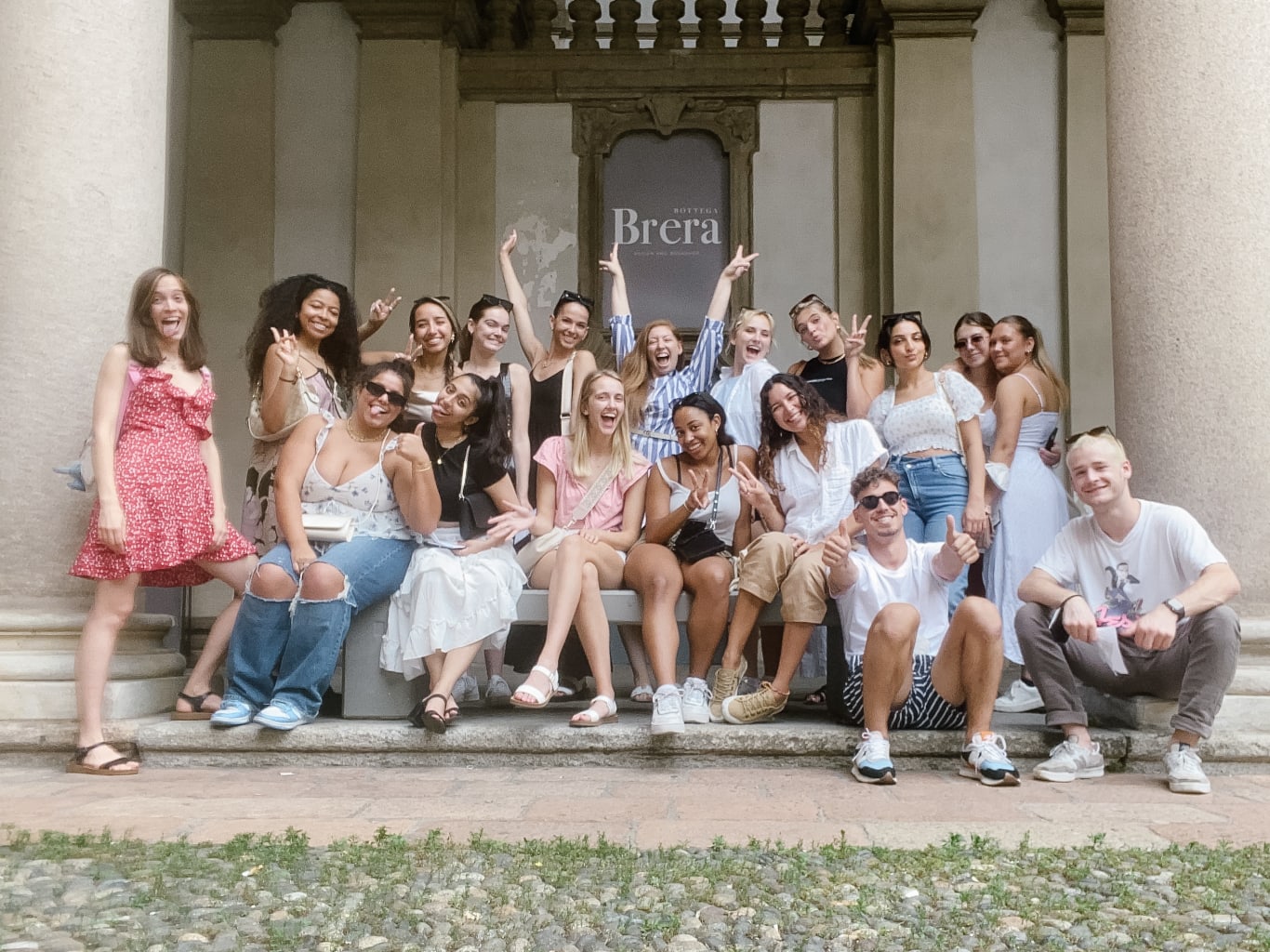This color daylight photograph captures an exuberant group of around 20 young people posing outside a stone building marked by grand sandstone or marble columns on both sides. The group includes both men and women of diverse backgrounds, with the majority being young women. They're seated and standing on and around a gray stone bench positioned in the entranceway, which steps lead up to, covered by the columns and a roof. Everyone is visibly excited, with broad smiles, thumbs up, peace signs, and playful expressions, contributing to the lively atmosphere. Behind the group, a rectangular sign with a gold trim reads "Brera" in white text. The foreground is a closely-fitted stone walkway, peppered with small green plants growing through the gaps, creating a vibrant, natural setting.